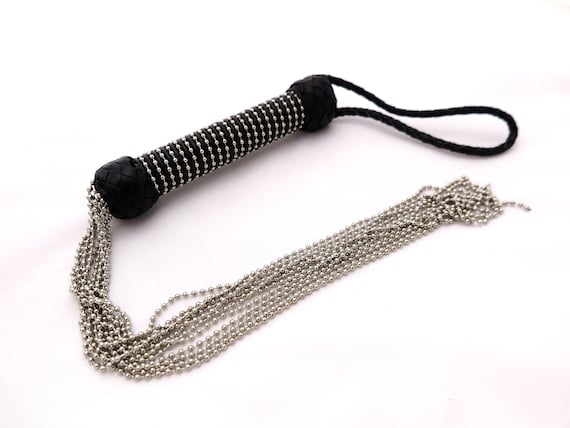The image depicts a studio-lit shot of a black leather whip, set against a stark white background. The whip features an intricately woven black leather handle, adorned with numerous thin silver chains, each made up of small metallic beads linked together. These chains wrap tightly around the handle, extending outward and curling towards the black leather rope at the other end. A black string attached to one end of the handle suggests it can be worn around the wrist for a secure grip. The overall appearance gives off a BDSM aesthetic, combining both functional and ornamental elements.